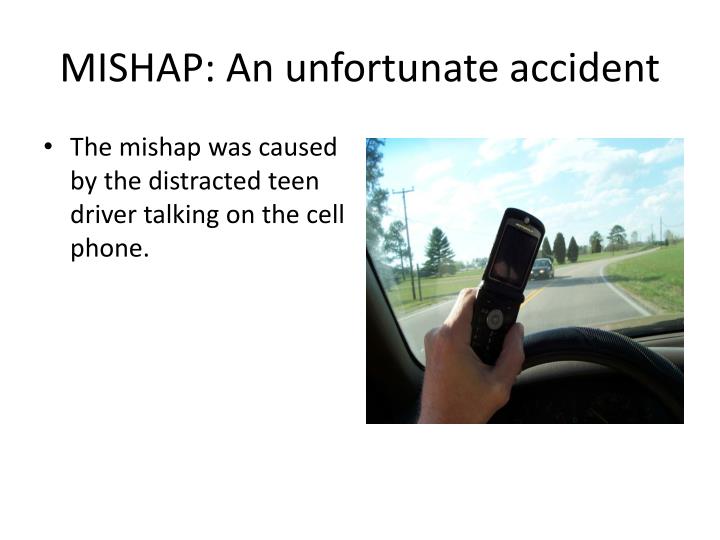The image is a PowerPoint slide with a white background, featuring both text and an illustrative image. At the top, centered, is the title "Mishap: An Unfortunate Accident," where "MISHAP" is written in capital letters and the rest in normal case. Below this title, on the left side, there is a bullet point with the text, "The mishap was caused by the distracted teen driver talking on the cell phone," written in black. To the right of this text is a detailed image taken from inside a car during the daytime. In the image, a hand on the steering wheel is also holding an open black flip phone. Through the windshield, the two-lane road ahead curves to the right and is marked with double yellow lines separating the lanes and white lines along the edges. Oncoming traffic is represented by a black vehicle in the opposite lane. The scene includes grassy areas on both sides of the road, a scatter of trees and a telephone pole on the left, and a cloudy sky overhead.